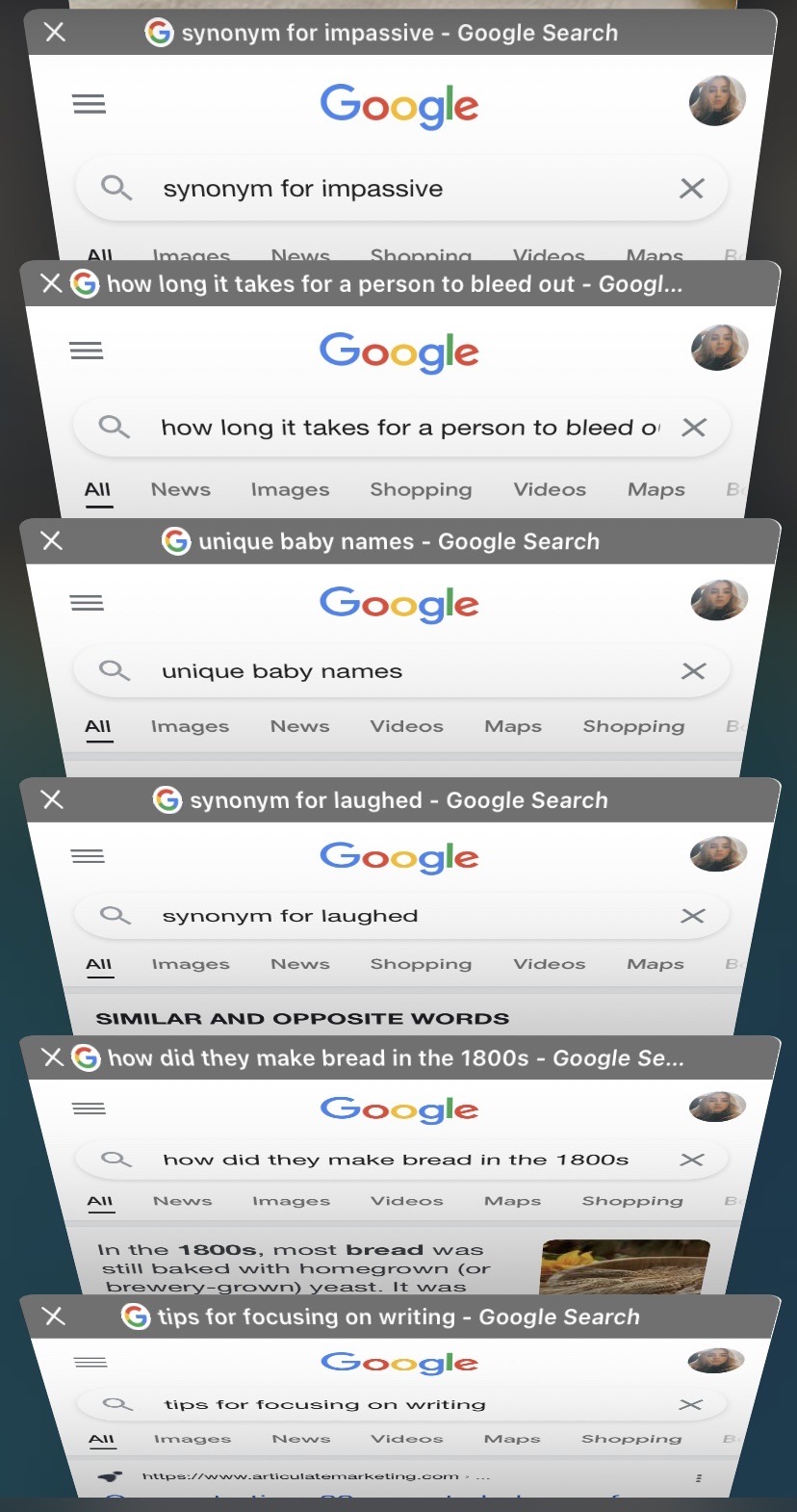The image showcases several different Google search windows, each representing a unique query. The first window displays a search for "synonym for impassive." The second window begins with "how long it takes for a person to bleed O" but the text is truncated. The third window searches for "unique baby names." The fourth window seeks a "synonym for laughed." The fifth window queries "how did they make bread in the 1800s?" The final window looks for "tips for focusing on writing."

At the top of each window is a medium grey strip with white, bold, and small font text indicating the search query. Next to each query in the grey area, there is a dash followed by "Google search." To the left of this text, there's the multicolored Google "G" symbol, encased in a white circular icon. Each window also features a light grey or white "X" in the upper left corner, offering the option to close the window.

To the right of each window is a user image, appearing to be a selfie of a woman with blonde hair. Above the search bar in every window, there are several categorized sections: "All," "News," "Images," "Shopping," "Videos," and "Maps," with "All" being highlighted and underlined in bold. On all windows except the first (where it gets cut off), you can see these section headers.

The iconic Google logo appears in every search window, composed of a blue "G," a red "O," a yellow "O," a blue lowercase "g," a green "L," and a red "E."